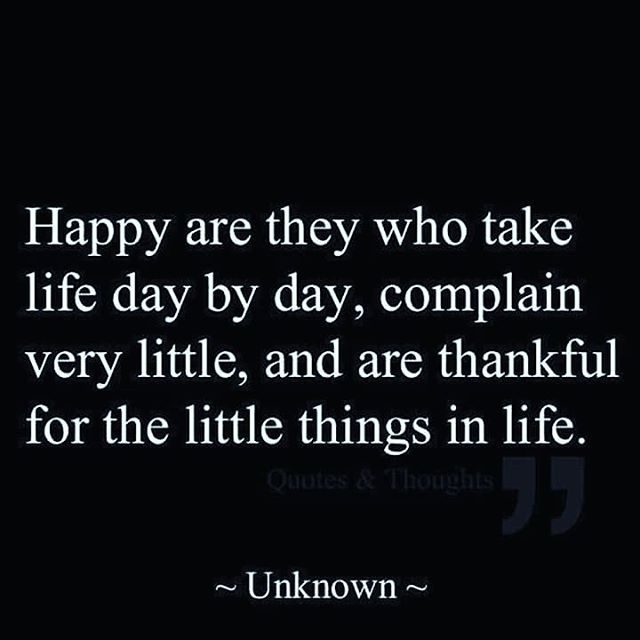The image features a simple, yet profound motivational quote presented in white text against a black background. The quote reads, "Happy are they who take life day by day, complain very little, and are thankful for the little things in life." Beneath the main text, very faintly in light gray, appear the words "Quotes & Thoughts," followed by a larger quotation mark. At the bottom center of the image, the word "Unknown" suggests that the author of the quote is anonymous. The design is minimalistic, with the central focus on the text itself, inspiring viewers to appreciate and simplify their perspectives on life.